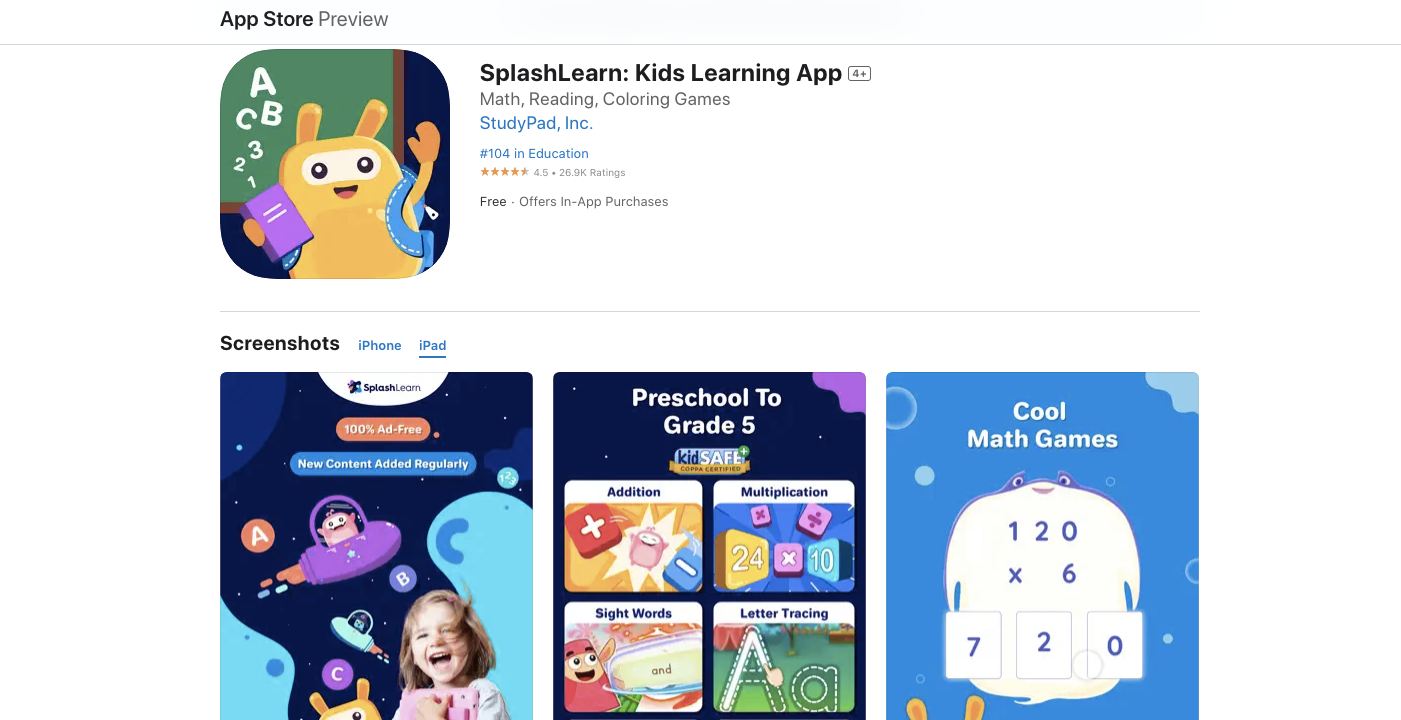**App Store Preview for "Splash Learn: Kids Learning App - Math, Reading, Coloring Games"**

The image showcases a clean, white background with "App Store Preview" written prominently at the top. Central to the illustration is a cute, cartoonish bunny character dressed in a yellow outfit, with distinct white facial markings around its black eyes. The bunny holds a purple book in one hand, sports a blue backpack, and waves cheerfully with its free arm. A chalkboard behind the bunny displays "ABC 123".

To the right of this central graphic, the app title "Splash Learn: Kids Learning App - Math, Reading, Coloring Games" is displayed in blue text. The app is ranked number 104 in the Education category.

Below this title, there is a line separating the app description from the screenshots section. The section is labeled for both iPhone and iPad devices, with "iPad" prominently underlined, indicating the selected preview. 

Three vividly animated screenshots follow:

1. The first screenshot features a smiling young girl with light skin and brown hair, set against a whimsical space background. The scene includes a small UFO and twinkling stars.
   
2. The second screenshot highlights educational content, labeled "Preschool to Grade 5." It displays various modules such as addition, multiplication, sight words, and letter tracing, each accompanied by cute animations of the bunny character. 

3. The final screenshot is labeled "Cool Math Games" and prominently features a cartoonish stingray. On the underbelly of the stingray are math problems like "120 x 6" and "720," all rendered in a playful, engaging manner.

This detailed depiction captures the essence of the "Splash Learn" app—a playful and educational tool designed to make learning fun for children.